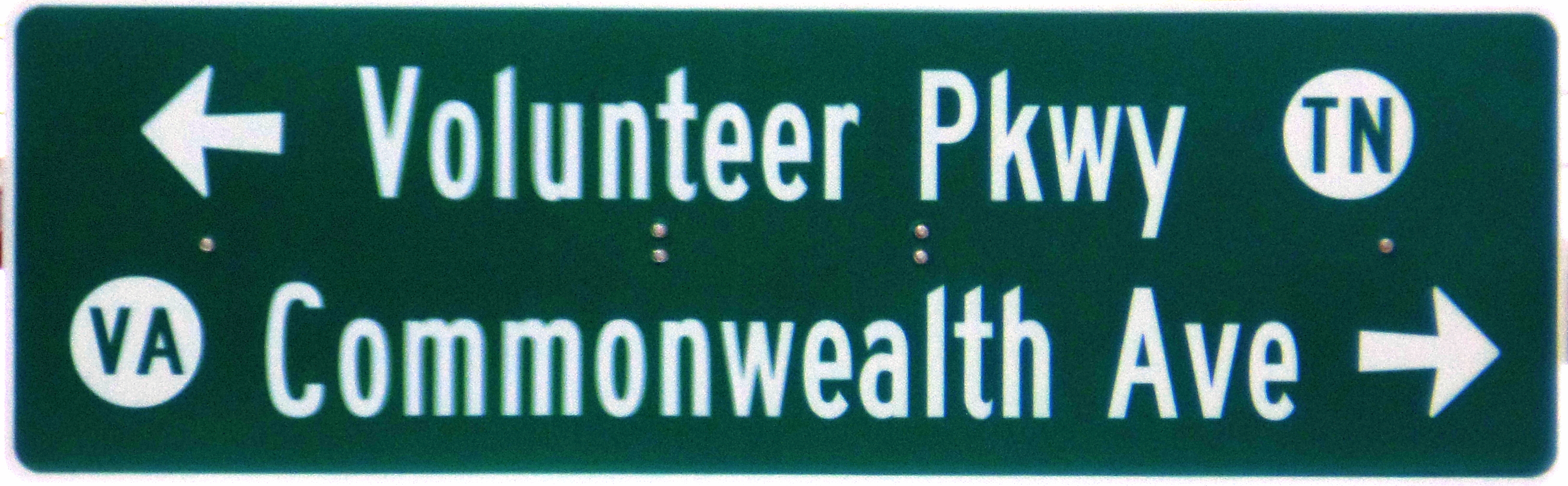The photograph presents a rectangular, green street sign with a white border, spanning approximately four times its height. Prominently occupying the frame, the sign provides directional information for motorists. At the top left section of the sign, the text "Volunteer Parkway" is clearly visible in white, accompanied by a left-pointing arrow, indicating the direction. Adjacent to this, the text "White Circle TN" is also displayed. 

Near the bottom of the sign, "Commonwealth Avenue" is inscribed in white text with a right-pointing arrow beside it to denote direction, and to the immediate left, a white circle with the letters "VA" can be seen, likely referring to a nearby Virginia route or locality.

The sign is affixed with metal bolts: two single bolts are located towards the left-center and right-center, respectively. Additionally, at the center of the sign, four bolts are arranged in pairs, securing it firmly in place. The image captures these details with slight blurriness but maintains overall clarity.